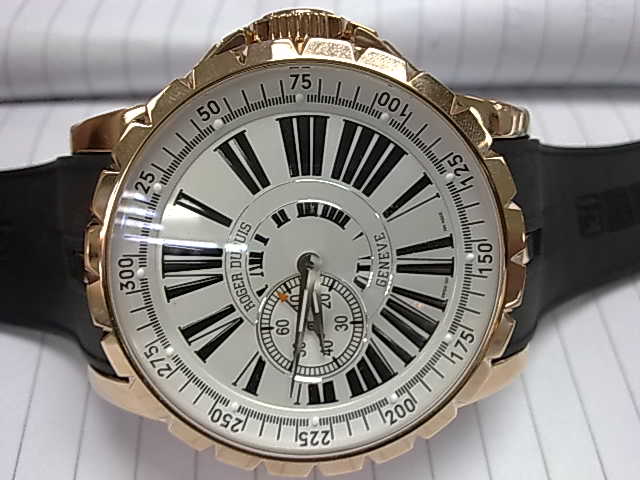The photograph features a close-up, horizontal view of a seemingly expensive watch. The watch boasts a black band and is set against an open composition-style notebook with lined pages. Its face is white, framed by a gold gear-shaped border. One notable feature is the large rounded knob positioned at the top of the watch. The outer edge of the bezel includes a measuring line with numbers ranging from 25 to 300, with 300 located on the left side. 

The watch face itself sports two black and white striped hands for telling time. Around the exterior, black Roman numerals are prominently displayed. Inside this main circle, an additional smaller circle can be found, also marked by Roman numerals. This inner circle contains a tiny secondary face with numbers ranging from 10 to 60. The text "Roger Deweese" is elegantly displayed near the top of the watch's face, while the word "Geneva" appears at the bottom. The watch is photographed on its side, requiring one to tilt the head to the left for a head-on view. The background reveals a white cloth with thin gray vertical lines that appear folded towards the back.